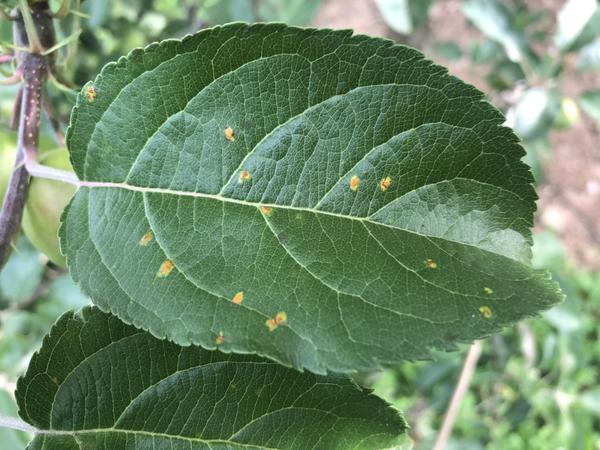A photograph captures a deep, dark green leaf prominently displayed at the center of the image, attached to a relatively thick, dark brown branch marked with light yellow speckling. The leaf is large and has serrated, notched edges, with a heavy, lighter veining running down its center, creating sections that give it a layered appearance with ridges. The leaf is marred by numerous yellow-reddish spots, likely indicative of disease or insect activity, numbering about a dozen in scattered pattern. To the left of this main leaf, there is an identical leaf that remains unblemished. The background reveals an out-of-focus array of additional green foliage and patches of dirt, suggesting a natural, possibly jungle-like outdoor environment.